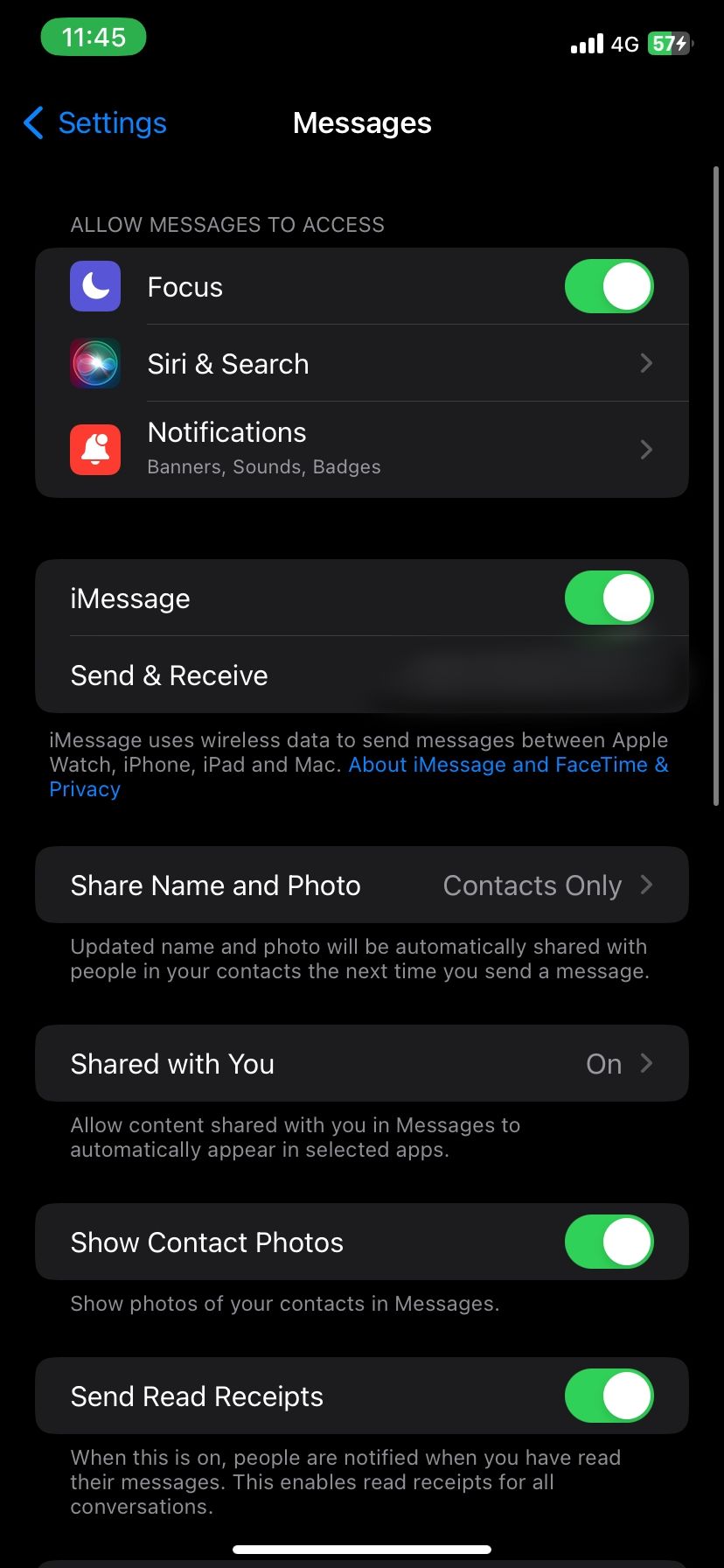Screenshot of a smartphone screen displaying the Messages settings tab. In the upper left corner, the time reads 11:45, and the device is connected to a 4G network with full signal strength and a battery charge of 57%. The user is in the "Messages" section under the "General" tab. 

At the top, the screen shows options allowing Messages to access various features: "Focus" is enabled, while the statuses for "Siri & Search" and "Notifications" are not specified. The iMessage feature is turned on, along with options to show contact photos and send read receipts, all indicated as active.

The interface has a black background with blue text. The word "Settings" is prominently displayed in blue at the top. Other blue text includes options and sections like "About iMessages and FaceTime & Privacy."

Below the "Notifications" section, additional options are visible such as "Send & Receive," "Share Name and Photo," "Shared with You," "Show Contact Photos," and "Send Read Receipts," all consistently detailed to give a comprehensive view of the screen's features and settings.